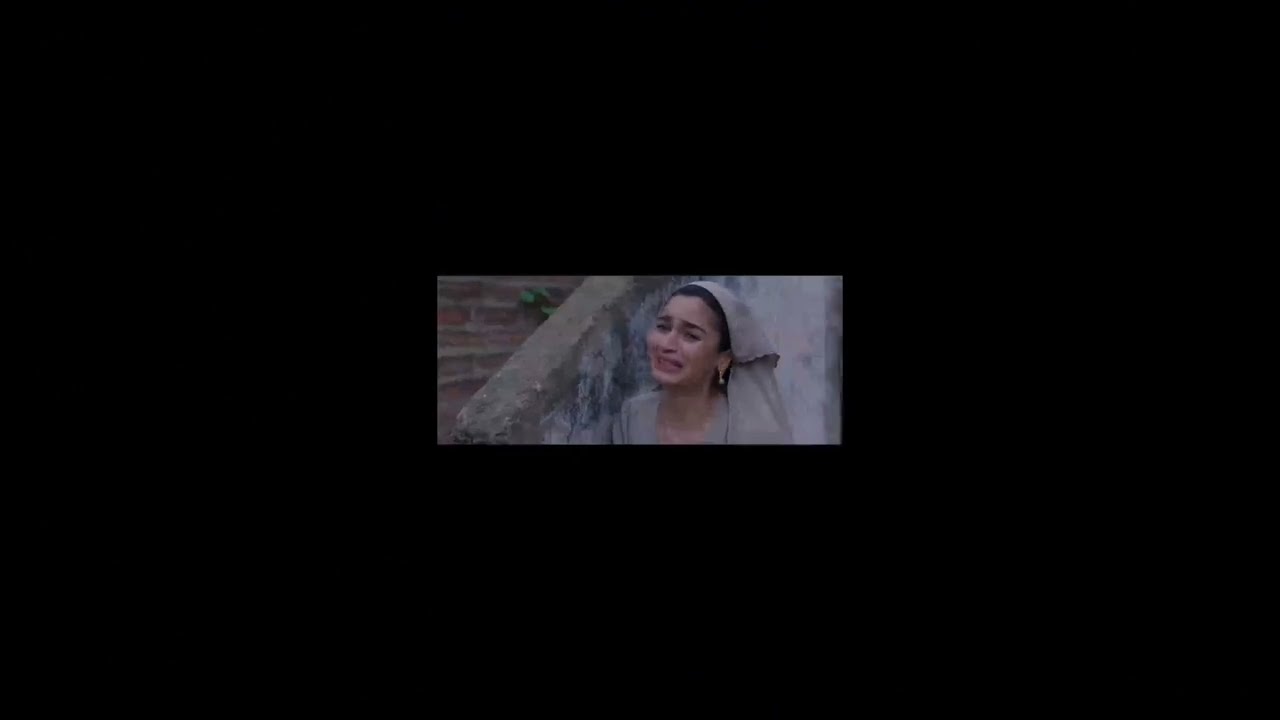The image is a horizontal rectangular scene with a predominantly solid black background and a smaller horizontal rectangle in the very center. In this central rectangle, the focus is on a young woman who appears to be crying profusely. She has dark hair pulled back and is wearing a brownish-colored veil that suggests she may be a nun or of Jewish heritage, and a matching tan dress that drapes over her shoulders. Her face reveals thick black eyebrows, high cheekbones pushed up by her intense crying, and squinted eyes, with her mouth open. She has a gold earring with a white pearl hanging from her left ear.

To the left of the woman, a brick wall with an old, painted, gray stone top is visible, accompanied by a stone railing with stairs ascending from the bottom left to the top right of the picture. Behind her, there appears to be a concrete wall, reinforcing the aged and textured background. The image, likely a screenshot from a movie scene, captures the woman's distress with meticulous detail.